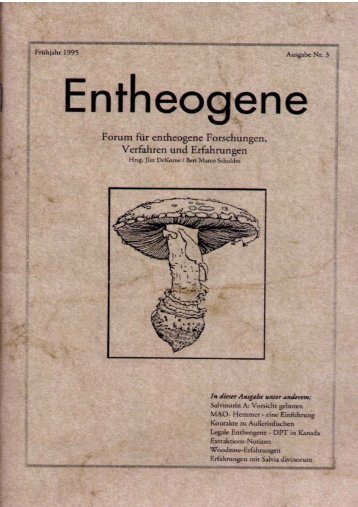The image depicts a beige, textured pamphlet or booklet titled "Entheogene," outlined by a black rectangular border. In the center of the cover, there's a detailed, hand-drawn illustration of a mushroom, showcasing its gills. Surrounding the illustration, there are various segments of text in black print, written predominantly in German, including phrases like "Form für Entheogene Forschungen Verfahren und Erbarungen." The pamphlet also features a date, "1995," in the upper right corner, along with "Nummer drei" to the right side. Additional text, difficult to decipher, is positioned both above and below the mushroom illustration, suggesting educational or informational content related to entheogens.